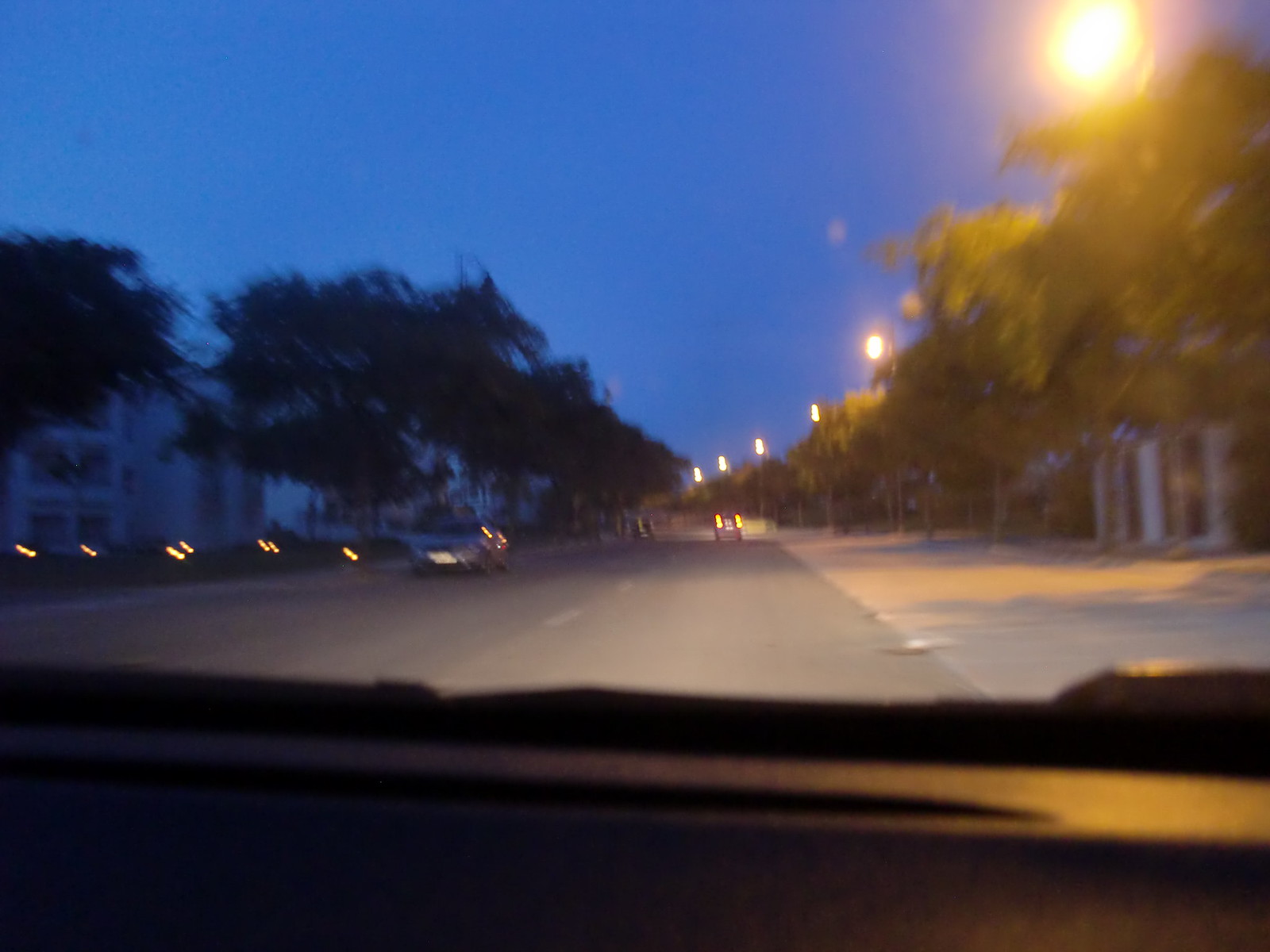This blurry nighttime image captures the viewpoint of a driver looking through their windshield. The scene reveals a car ahead with three lit brake lights, its own red taillights visible in the dim surroundings. To the sides, we can glimpse several greenish trees, with one displaying a faint patch of white on its trunk. A silver sports car is either driving by or parked, adding a touch of metallic sheen to the scene. To the left, there appears to be a house or a complex clad in white, set back slightly from the road. Below this structure, a sidewalk or an additional lane is slightly more illuminated, showcasing a contrast in the pavement. Additionally, an intense glare from a presumed streetlight occupies the upper right corner of the image, cutting through the darkness of what seems to be a late evening, likely around 7 or 8 PM.